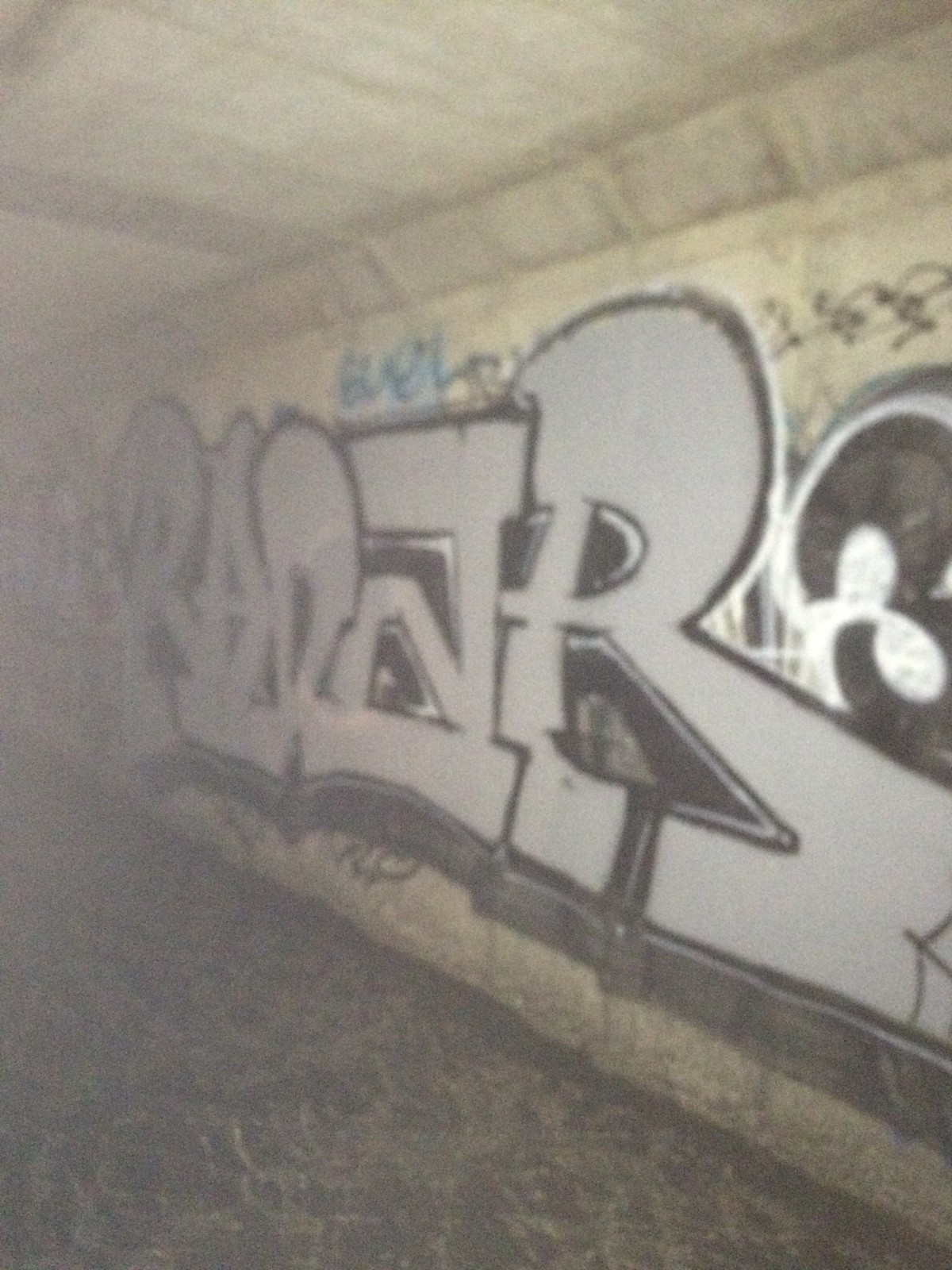The photograph captures the interior of a concrete tunnel, likely a sewage or drainage tunnel, as suggested by what appears to be water flowing on the floor, reflecting light in a wavy pattern. The tunnel's walls and ceiling are a beige color. Dominating the wall is a large piece of graffiti that stretches from the floor to the ceiling. This graffiti, marked by exaggerated and artistically rendered letters, seems to spell "RADNTR" in grey font, accented with black outlines and black shadows within the letters. Above this prominent graffiti, there's a small bit of blue graffiti, and to the right, a black number "3" with a white outline is visible. The tunnel wall also bears older, smaller graffiti, which is out of focus in the photo.